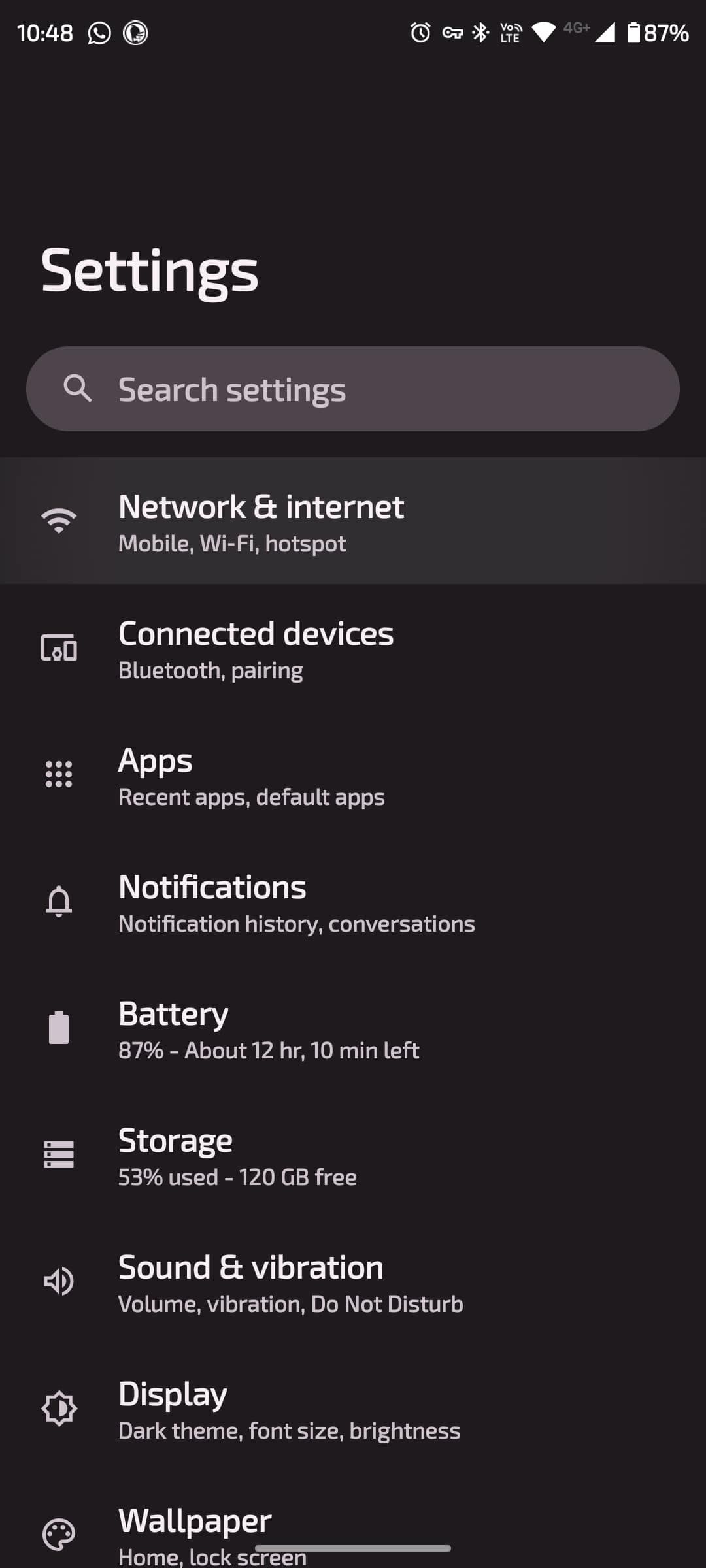The image background is black, indicating it's a screenshot likely taken from a cell phone. In the upper left corner, the time is displayed as 10:48. On the upper right, the battery life reads 87%. Just below, the word "Settings" appears in white text. A horizontal oval-shaped area shows a magnifying glass icon followed by the phrase "Search settings."

The list below comprises various settings categories:
1. **Network & internet:** Sub-options include Mobile, Wi-Fi, Hotspot.
2. **Connected devices:** Sub-options include Bluetooth and Pairing.
3. **Apps:** Sub-options include Recent apps, Default apps.
4. **Notifications:** Sub-options include Notification history and Conversations.
5. **Battery:** Displays 87% remaining with an estimated 12 hours and 10 minutes of usage left.
6. **Storage:** Indicates 53% used, with 120 gigabytes free.
7. **Sound & vibration:** Sub-options include Volume, Vibration, Do Not Disturb, with a speaker icon to the left.
8. **Display:** Sub-options include Dark theme, Font size, Brightness.
9. **Wallpaper:** Specifies options for Home and Lock screen.

Each category is clearly delineated, with corresponding options making it easy to navigate various settings on the device.